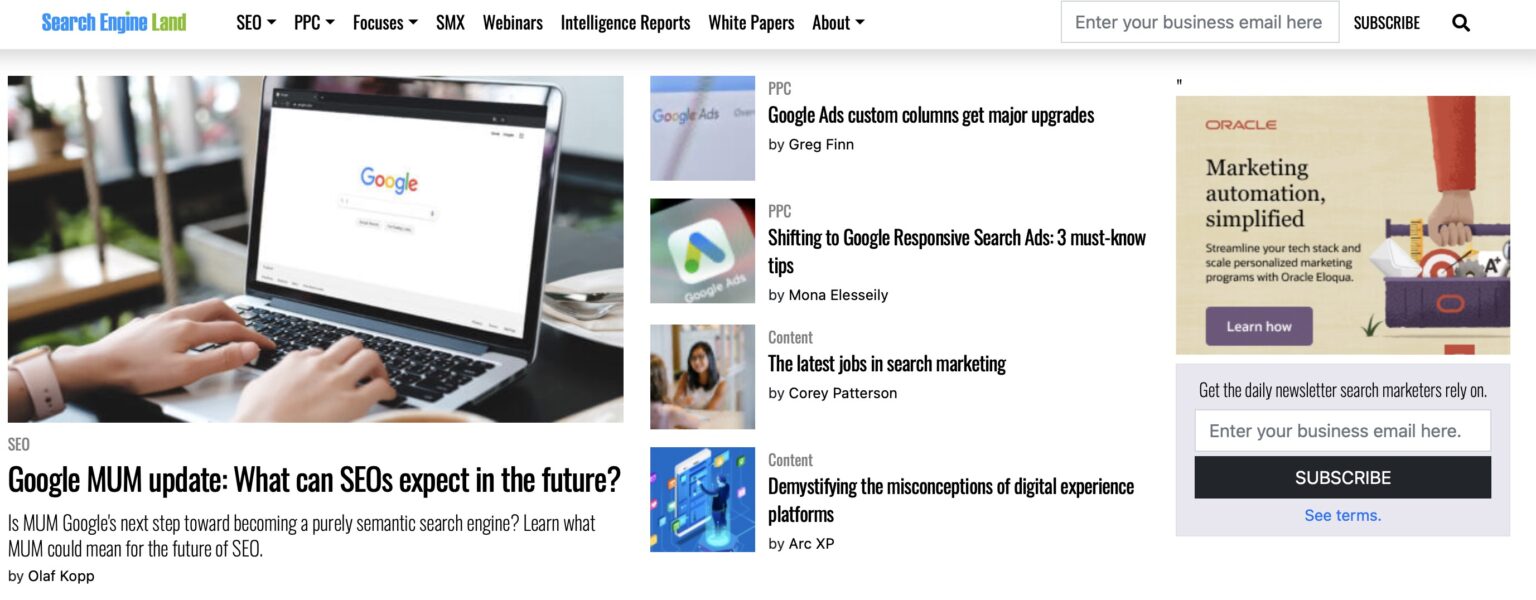The image captures a screenshot of the "Search Engine Land" website, presented in a format that is approximately four times wider than it is tall. At the very top of the webpage, a white background supports the main navigation menu. On the left side of this bar, the company logo features the words "Search Engine" in light blue followed by "Land" in lime green.

To the right of the logo, the navigation menu includes the following categories in black font: SEO, PPC, Focuses, SMX, Webinars, Intelligence Reports, White Papers, and About, with drop-down arrows accompanying the first three and the last category. Towards the far right of the menu, there is a text box prompting users to "Enter your business email here," followed by a black, bold, and capitalized "SUBSCRIBE" button. Adjacent to the subscribe button is a magnifying glass icon, indicating the search function.

The main content area beneath the menu is dominated by a large banner image showing two hands on a silver laptop, angled such that the screen faces about the seven o'clock position. Below this banner, the headline reads, "Google MUM Update: What Can SEOs Expect in the Future?" accompanied by a descriptive sentence. To the right of the main article, there is a vertical arrangement of four additional articles, hinting at a well-organized and content-rich webpage.